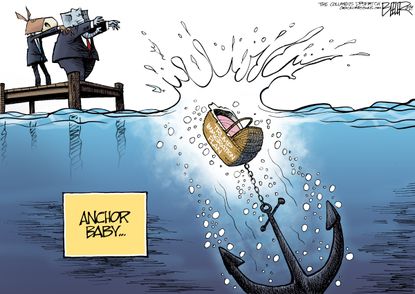The image is a detailed political cartoon set on a small, wooden pier over clear blue water. Two figures in suits stand on the pier's edge, depicted as anthropomorphic animals to symbolize political parties: one has the head of a donkey, is skinny, and wears a gray suit with a blue tie; the other has the head of a bulky elephant, is more robust, and is dressed in a gray suit with a red tie. Both figures appear to be sleepwalking off the end of the pier, seemingly oblivious.

Below them, a bassinet tied to a heavy anchor has just splashed into the water. The bassinet, which contains a pink blanket, is being dragged toward the ocean floor by the black anchor. A label with a yellow background on the left side of the image reads "Anchor Baby." Additionally, the anchor bears another label that says "Trump Immigration Plan."

In the upper right corner of the image, there is a title and a signature, though they are small and unclear, potentially accompanied by a barely legible website URL. The blue water beneath the pier contrasts sharply with the wooden structure and the dramatic splash created by the submerged bassinet, drawing attention to the central theme of the cartoon.